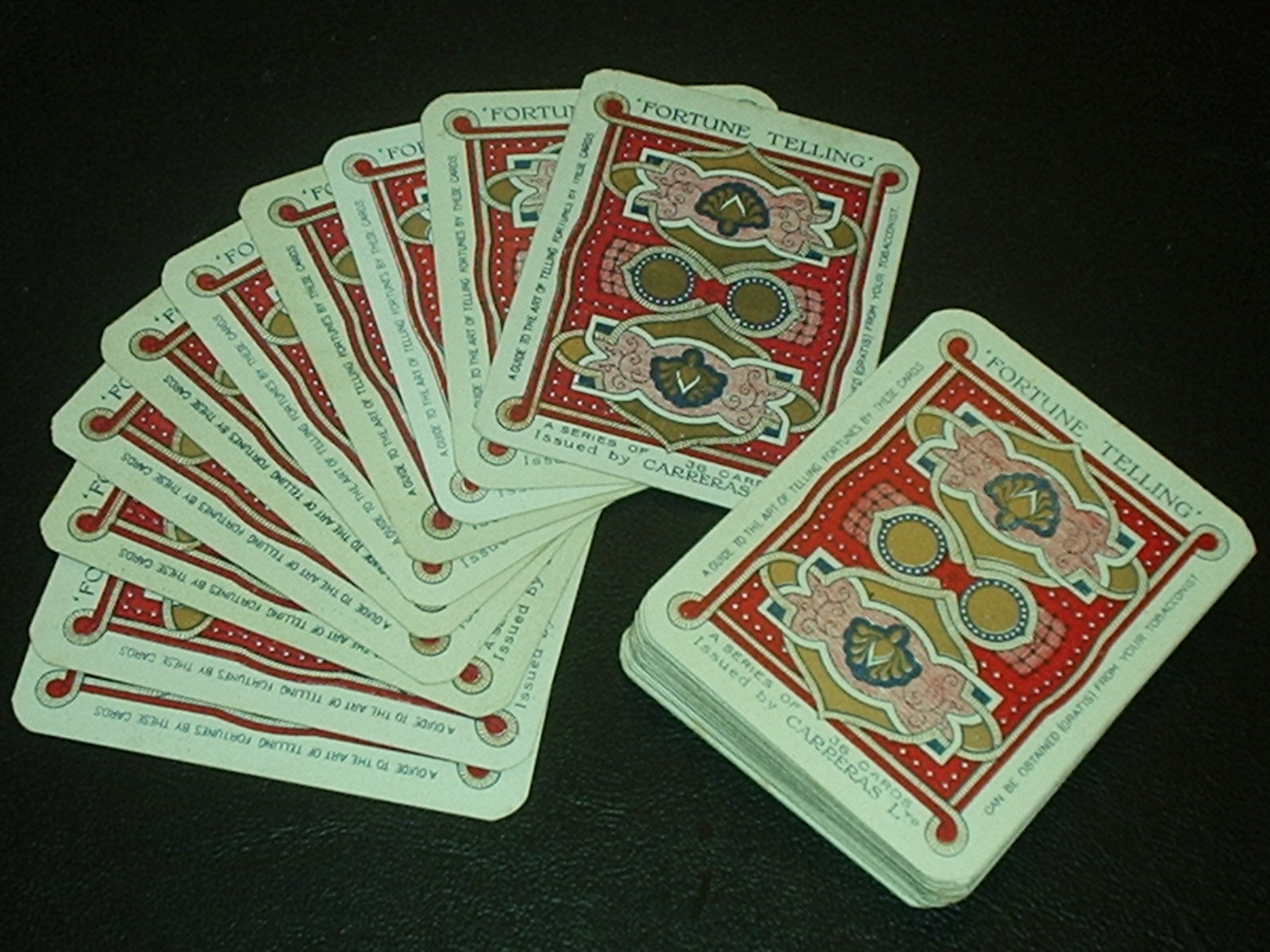The image features a black-painted, rough-textured table in the background. On the right side of the table, there is a neatly stacked pile of fortune-telling cards. To the left of the stack, there are ten fortune-telling cards arranged side by side, resembling a spread of playing cards in a hand. The design of the cards is distinctive and detailed. At the top of each card, the words "Fortune-Telling" are prominently displayed. Below this text, a vertical red rectangular design with a white border houses rows of horizontally aligned white dots. Across the red border, a gold symbol, reminiscent of a badge, features a pink motif overlaid with an intricate gold and blue seashell-like symbol. Beneath this design, two round golden elements are situated. At the bottom of each card, the text reads: "A series of J6 cards issued by Corebus."